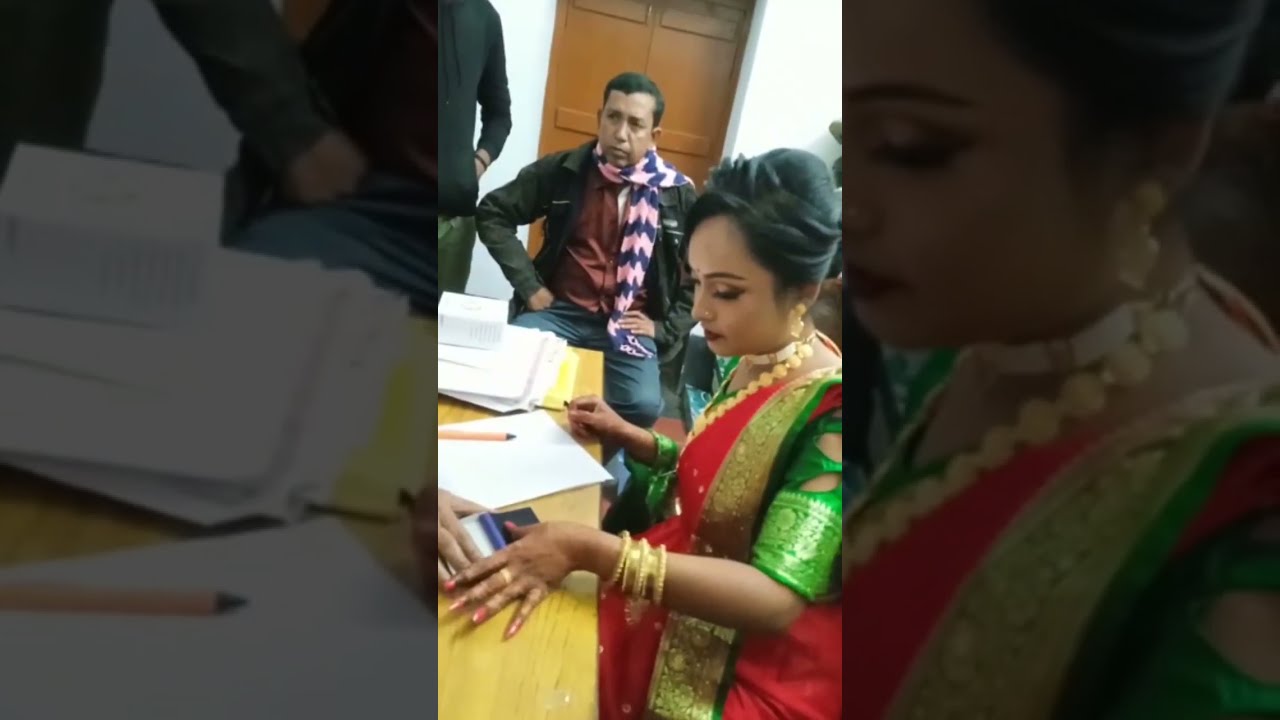The image depicts an elaborately dressed Indian woman, adorned in a bright red sari with gold and green accents, sitting at a light brown wooden table in an office setting. Her black hair is styled into a bun, and she displays an array of gold jewelry, including bangles, a thick necklace, and earrings. Her nails are painted red. She appears to be pressing her thumb into an ink pad, possibly for a fingerprint verification, amidst stacks of white paper on the table. Beside her, on the table, rests a pencil and what may be a calculator. Behind her, the background features a brown door and a white wall, with two men visible. One man, partially cut off, is wearing a black hoodie and olive green pants, while the other, seated at the far end of the table, is dressed in blue jeans, a leather coat, a burgundy shirt, and a scarf with pink and blue stripes. The atmosphere suggests an official or bureaucratic process taking place.